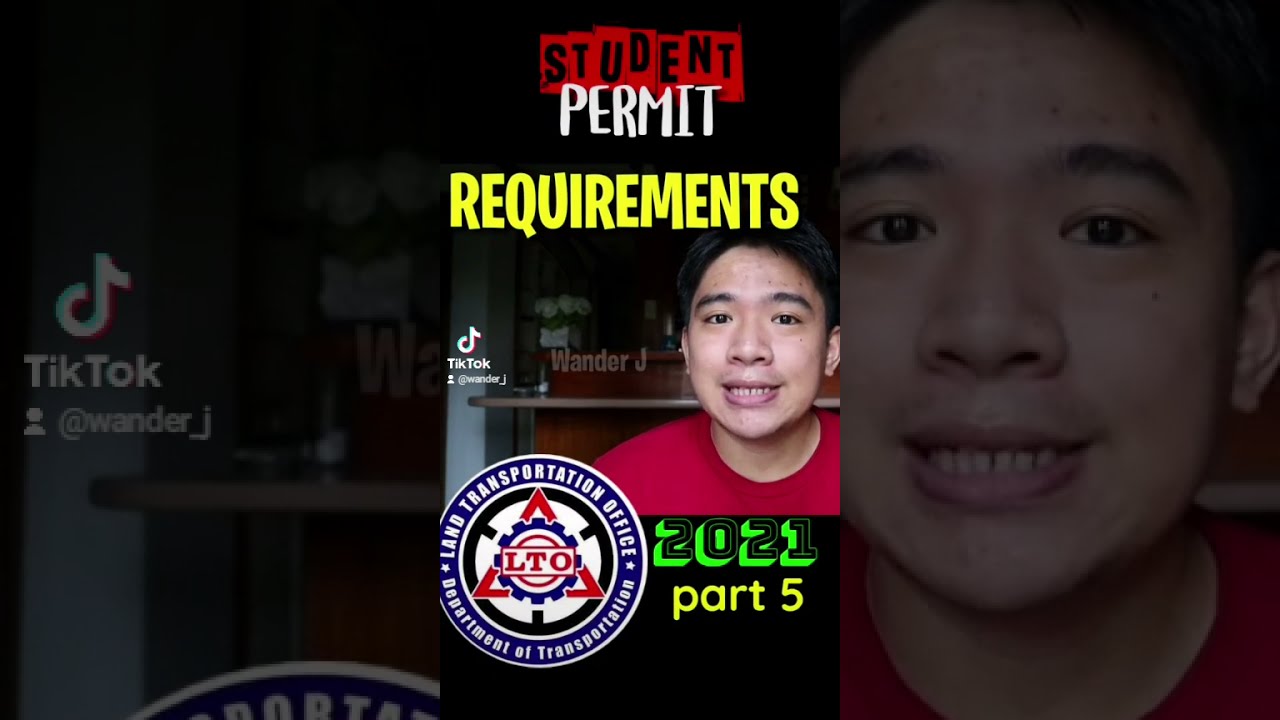The image is vertically divided into three sections. The central section features a screenshot from a video, showing a young boy, possibly of Asian descent, with short black hair, dark-colored eyes, and light brown skin. He is wearing a red t-shirt and his mouth is open, revealing his lower teeth. Text above him reads "Student Permit Requirements" in a combination of red, white, and gold lettering on a black background. At the bottom, in green and yellow text, it states "2021 Part 5". To the left of the boy, there's a TikTok icon labeled "@wonder_jay". Adjacent to the TikTok icon is a circular logo featuring a triangle with a gear inside it, and the letters "LTO". The logo is labeled "Land Transportation Office, Department of Transportation" around its perimeter. The outer sections of the image are enlarged and darkened close-ups of the boy's face and the TikTok icon, creating a cohesive background.